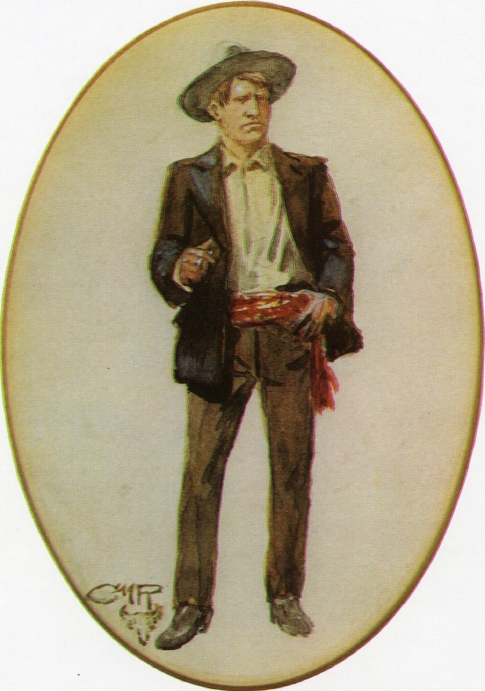This is an oval-shaped painting with a white background, showcasing a detailed portrait of a man who embodies the essence of a cowboy. The man is dressed in a black jacket over a white button-up shirt, paired with brown slacks and presumably nice shoes or cowboy boots. A distinctive red cloth belt with a fringe hanging down adorns his waist, where his left thumb is looped through. His right hand holds a cigarette, adding to his rugged demeanor. He has brown hair and is wearing a smaller cowboy hat with a flipped-up brim. His head is tilted slightly to the right as he gazes directly at the viewer. In the lower left portion of the painting, there are letters, either "CMR" or "CHR," alongside a stamped insignia of a steer's head, enhancing the western theme. The painting prominently features shades of tan and brown, accentuated by the red belt, capturing a classic and nostalgic cowboy image.